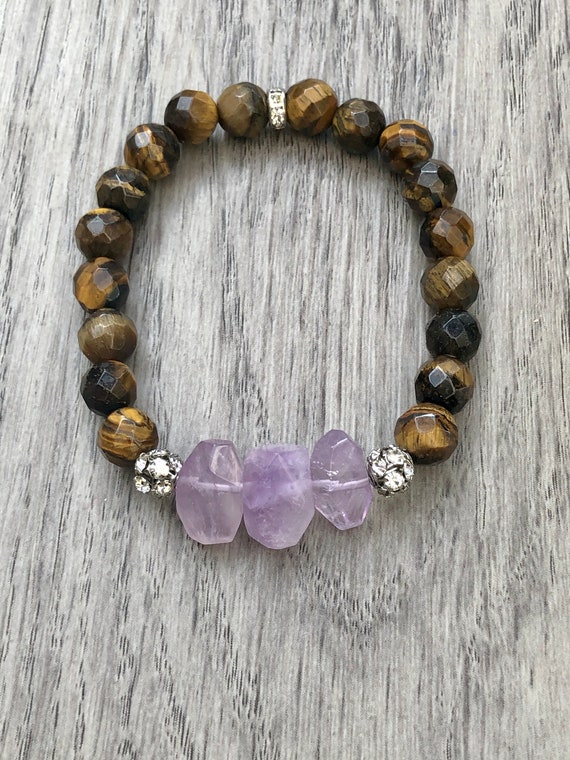This vertically aligned rectangular image captures a close-up of a beaded bracelet placed on a light gray wooden surface with visible darker gray grains running through it. The bracelet features round, shiny, and slightly irregular wooden beads, predominantly dark brown in color. At the center, a small silver nugget or metal piece separates two of the beads. Further down, the bracelet is adorned with three large, light purple stones, possibly amethysts, which are irregularly shaped but closest to oval forms. On either side of this cluster of stones, there are small, crumpled-looking silver or metal balls. The overall aesthetic of the bracelet exudes a handcrafted charm, with its earthy tones and textured details, suggesting a modest value range, perhaps between $30 to $50.